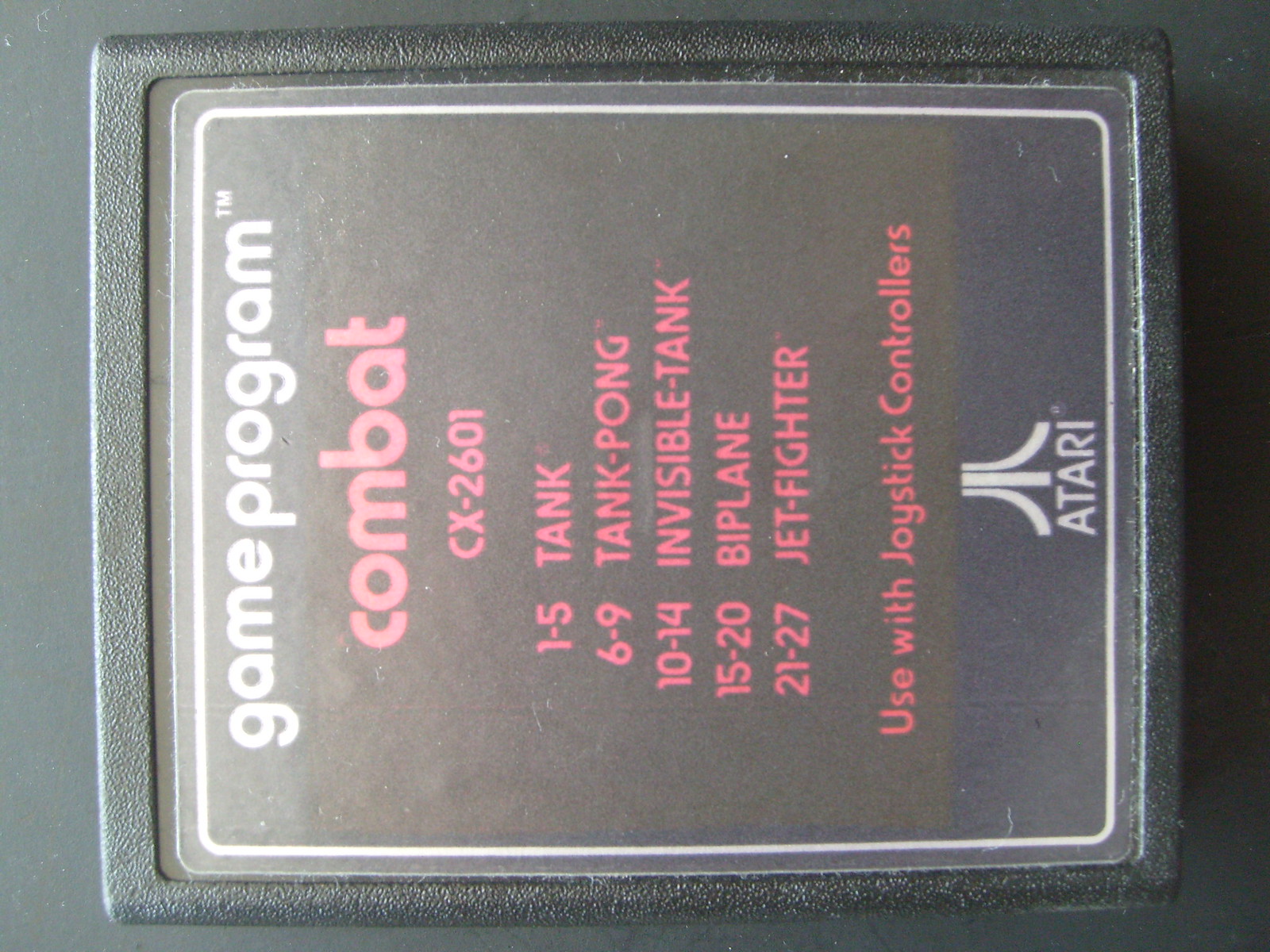This photograph showcases an Atari video game cartridge lying on its side on a black surface. The cartridge itself features a black textured border and bears a black sticker that covers the rectangular item. At the top of the sticker, in white lettering, it reads "Game Program," followed by the title "Combat" in prominent red letters. Below the title, there are additional details, including numbers and descriptions that likely correspond to game statistics or instructions. Further down, in red letters, the text advises "Use with joystick controllers." At the bottom of the sticker, the iconic white Atari logo is displayed. This image vividly captures a nostalgic piece of video game history, specifically an Atari game cartridge designed for use with joystick controllers.